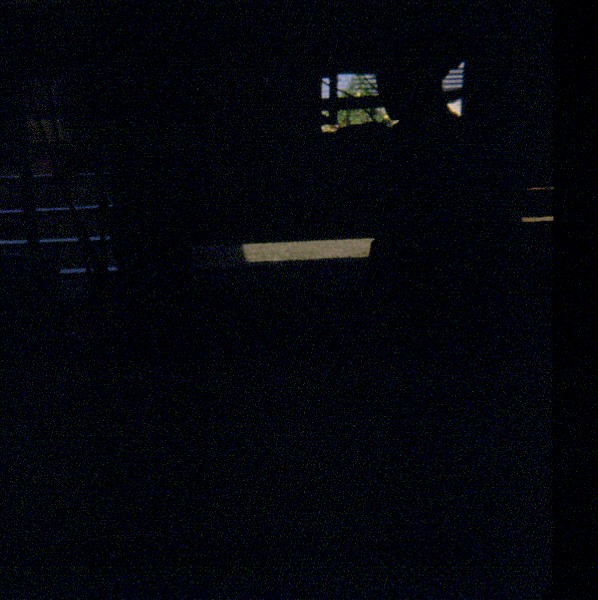In this predominantly black square image, the scene appears to be set inside a dark room where minimal light illuminates certain elements. The bottom half of the image is entirely black, creating a stark contrast with the top half, which features scattered flecks of light. At the center, slightly above the midpoint, there’s a small, landscape-oriented rectangle with an olive green or brown hue, possibly depicting a ground surface lit by some indirect light. The highlight of the top right corner is an open window adorned with Venetian blinds. This window allows glimpses of the outside, revealing a green tree against a faintly blue sky. The blinds, predominantly horizontal, show a thicker, seemingly stuck section towards the middle. 

Additionally, there’s a faint delineation of blue lines on the left side of the image, spread across different sections. Prominently, the silhouette of a human head is visible in front of the window, capturing the outline from the neck up to the forehead, angled towards the right side. Despite the detailed elements, the overwhelming darkness engulfs the scene, making most features appear as monochromatic silhouettes. The interplay of sparse light and deep shadows creates an enigmatic atmosphere.